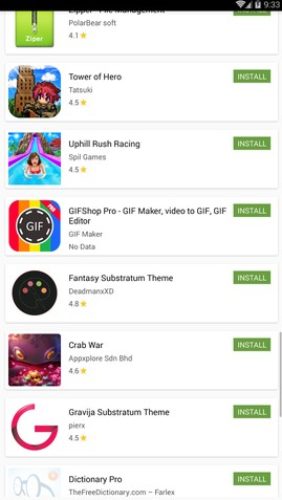In the provided phone screenshot, we observe a detailed arrangement of various apps available for installation. The image captures the phone's home screen at 9:33 AM, indicated by the time display at the top right corner. Adjacent to the time display, from right to left, are icons indicating app notifications – specifically, the Facebook logo, a strong phone signal at three out of four bars, and a fully connected Wi-Fi signal.

Moving lower, on the left side, we see a vertical list of apps. The first app's name is partially obscured, but it features a green square logo with the word "Zipper" prominently displayed. Following this is the game titled "Tower of Hero," represented by a hero in front of a tower. Continuing downwards, we find "Uphill Rush Racing." The next entry is a utility app named "GIF Shop Pro: GIF Maker, Video to GIF, GIF Editor," noted for its comprehensive GIF creation and editing capabilities.

Below this utility, there is an app called "Fantasy Substratum Theme," possibly for customizing the phone's appearance. This is followed by another game, "Crab War," and subsequently, another theme customization app named "Gravity Substratum Theme." The final app listed, found at the very bottom, is "Dictionary Pro," likely offering comprehensive dictionary functions.